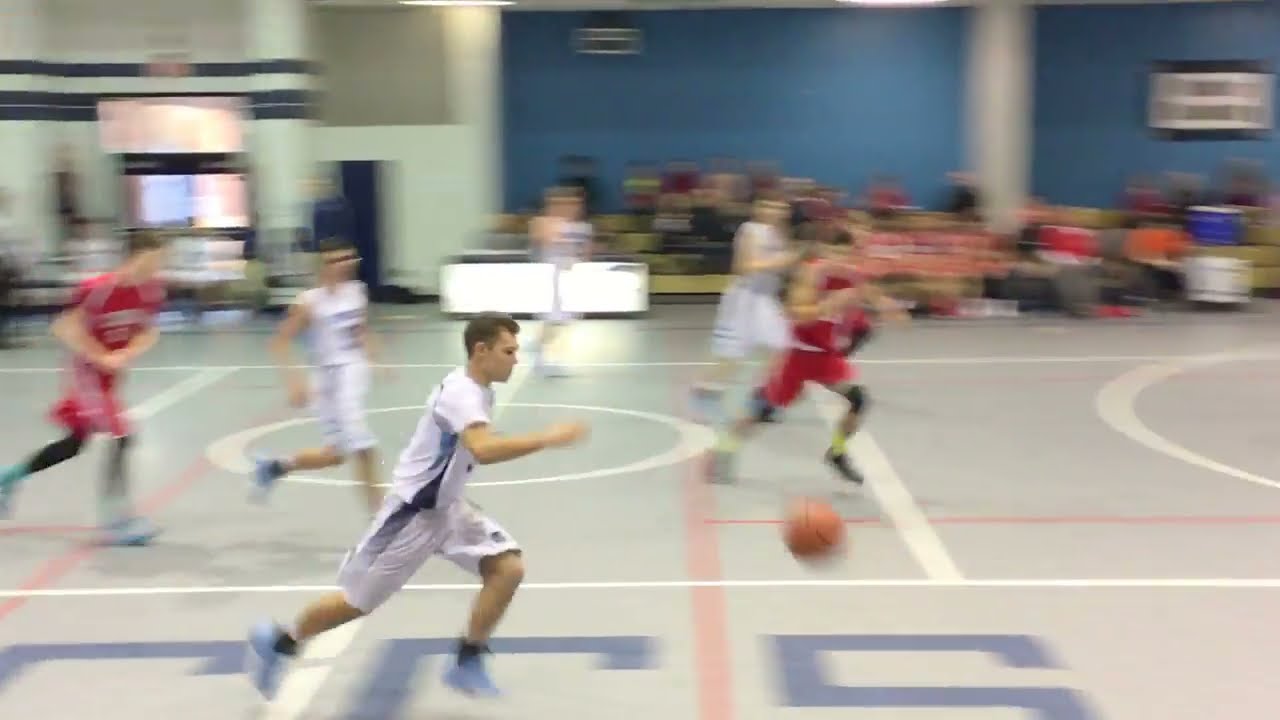In this dynamic and slightly blurred photograph of an indoor basketball game, the action is centered around a fast break by the team dressed in gray and blue jerseys with blue sneakers. At the forefront, a man in gray and blue is charging across the center court, chasing after a loose basketball that hovers tantalizingly close but just out of his reach. Trailing behind him are two men in red jerseys and two more in gray, all sprinting in the same direction to either advance the play or defend against it. The court itself is a distinctive gray with red and white striping, and the faint outline of an 'S' is visible on the glossy floor. In the background, the gymnasium extends into a darker blue wall to the right and a lighter gray wall to the left. Wooden bleachers are visible, with a few indistinct spectators seated, adding to the atmosphere. A doorway leading out of the gymnasium is seen in the top left corner, while an indiscernible sign captures the upper right corner. The fast-paced scene encapsulates the intensity and excitement of the game unfolding in a clearly active and energetic environment.